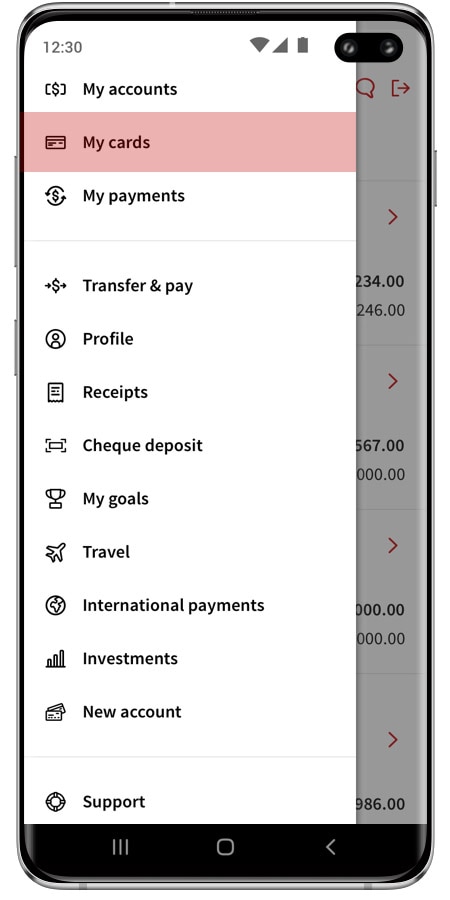The image captures the screen of a cell phone, showing a comprehensive array of app navigation icons. In the top left corner, the time is displayed as "12:30." On the top right corner, there are status icons for wireless signal, cellular connection, and battery level.

The main portion of the screen is dedicated to various app icons and their corresponding labels, arranged in a vertical list:
1. **My Accounts**: Represented by a dollar sign icon.
2. **My Cards**: Illustrated with an icon of a card.
3. **My Payments**: Depicted by a picture of two circular arrows surrounding a dollar sign.
4. **Transfer and Pay**: Shown with a dollar sign flanked by two arrows.
5. **Profile**: Indicated by a circle enclosing an image of a person.
6. **Receipts**: Represented by an icon of a piece of paper with writing on it.
7. **Check Deposit**: Illustrated with a picture of a check.
8. **My Goals**: Depicted by a trophy icon.
9. **Travel**: Shown with an airplane icon.
10. **International Payments**: Represented by a globe icon.
11. **Investments**: Indicated by an image of several bar graphs.
12. **New Account**: Depicted by an illustration resembling two cards together.
13. **Support**: Shrunk with a life preserver icon.

Each icon is illustrative of the specific service it represents, providing a user-friendly navigation interface for managing various financial and lifestyle services.